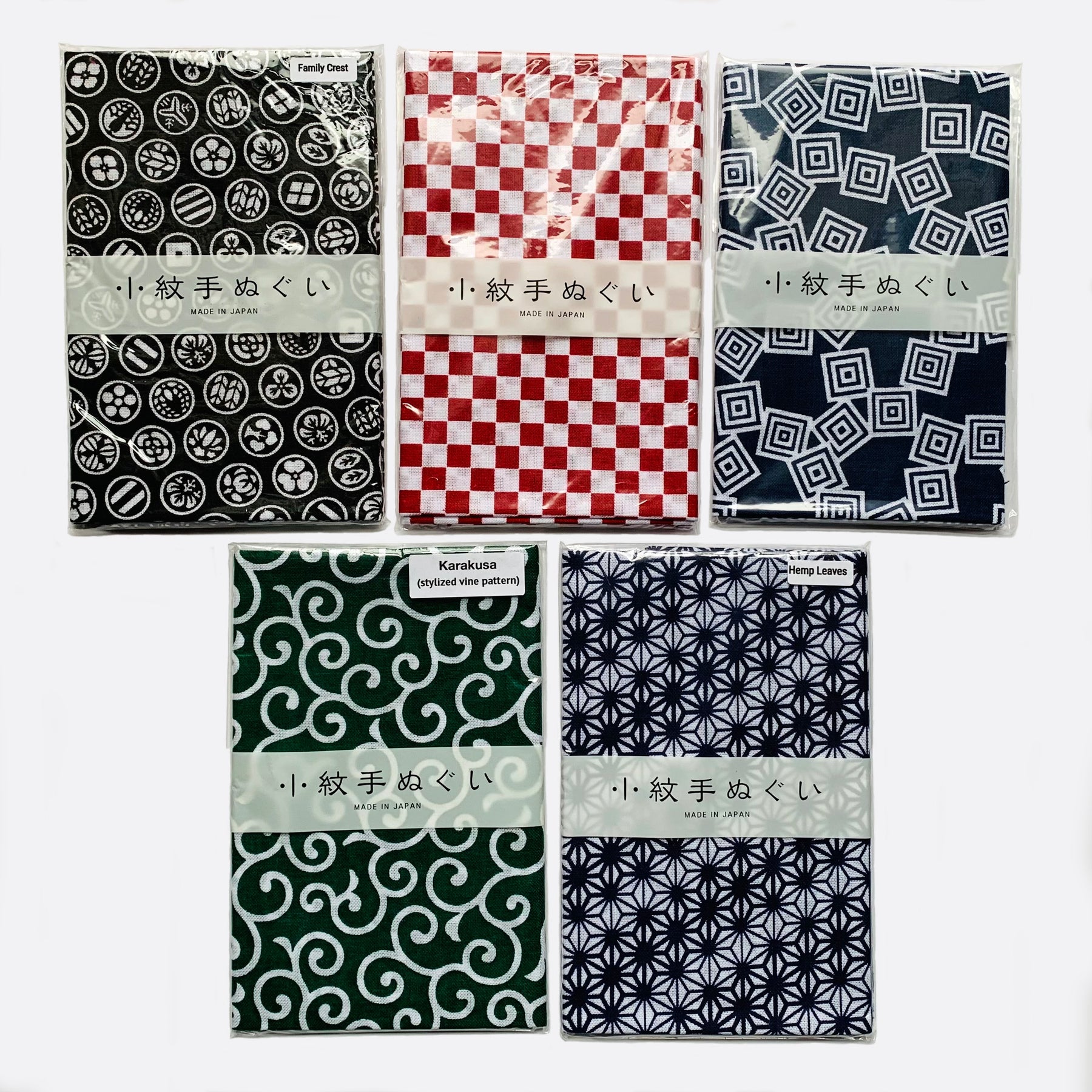This image showcases five individually packaged cloth pieces, each wrapped in a clear plastic bag, likely intended for a retail or commercial setting such as online shops, catalogs, or websites. The background is a clean light gray, emphasizing the vivid patterns on the fabrics. The products are arranged in a rectangular layout with three pieces on the top row and two on the bottom. 

The top left features a black fabric adorned with white circles, each containing various crests, including flowers, balls, and other intricate designs, labeled "Family Crest." The top center displays a red and white checkerboard pattern. The top right shows a blue fabric with white square shapes forming a detailed geometric pattern. 

On the bottom row, the left cloth is green with an intricate pattern of white curved lines, identified as "Karakusa Stylized Vine Pattern." The bottom right fabric is white, decorated with black floral and star-like designs, referred to as "Hemp Leaves." The packaging indicates the products are "Made in Japan," both in English and Japanese characters.